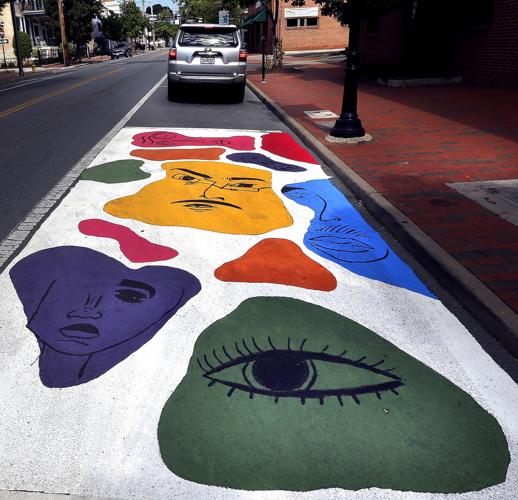This captivating image depicts a vibrant mural painted on a white surface along a brick-colored sidewalk on a typical street. The mural features an array of colorful, freeform shapes in hues of purple, green, red, orange, yellow, and blue, each with intricate designs painted in black. Prominent elements include a large purple face with one eye, a green rock-like form with a pronounced eye and eyelashes, a yellow shape with a man's face donning a mustache and glasses, and a bright blue blob with a nose, mustache, and lips. The background is dominated by a gray Subaru or Toyota SUV parked along the street, adding to the urban setting. Distinct white lines on the road separate the parking from the traffic lane, further highlighting the mural's striking presence in the scene.